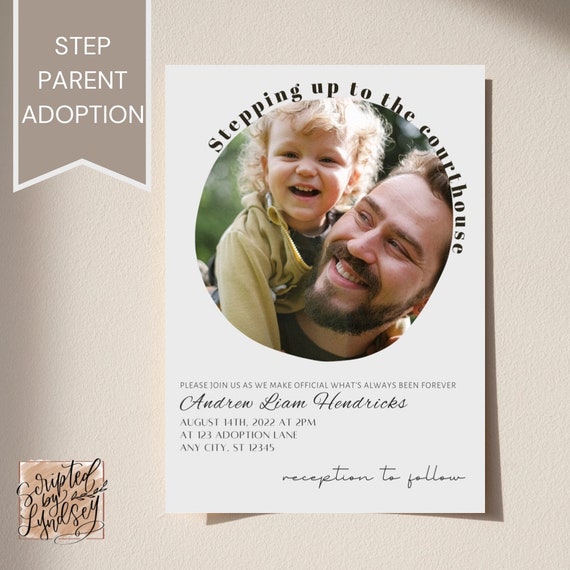This is a detailed photograph of an announcement card for a step-parent adoption. The card is a regular thin 8x10 white piece of paper hanging on a beige wall. In the upper left corner, a banner with a bookmark shape reads "Step-Parent Adoption." The central focus of the card is a circle containing an image of a bearded man with short brown hair, who appears to be in his 30s. Mounted on his back is a smiling child with short curly blonde hair, wearing a green hoodie or sweater. They both seem to be outdoors.

Above the circle, in black text, the card reads: "Stepping Up to the Courthouse." Below the image, it continues with: "Please join us as we make official what's always been forever." Further down, in black cursive, the name "Andrew Liam Hendricks" is written. The details of the event follow: "August 14, 2022, at 2 p.m., at 123 Adoption Lane, Any City, ST 12345." Lastly, there's a note indicating a reception to follow. This heartfelt flyer is a beautiful invitation to witness a meaningful moment in the lives of a family.